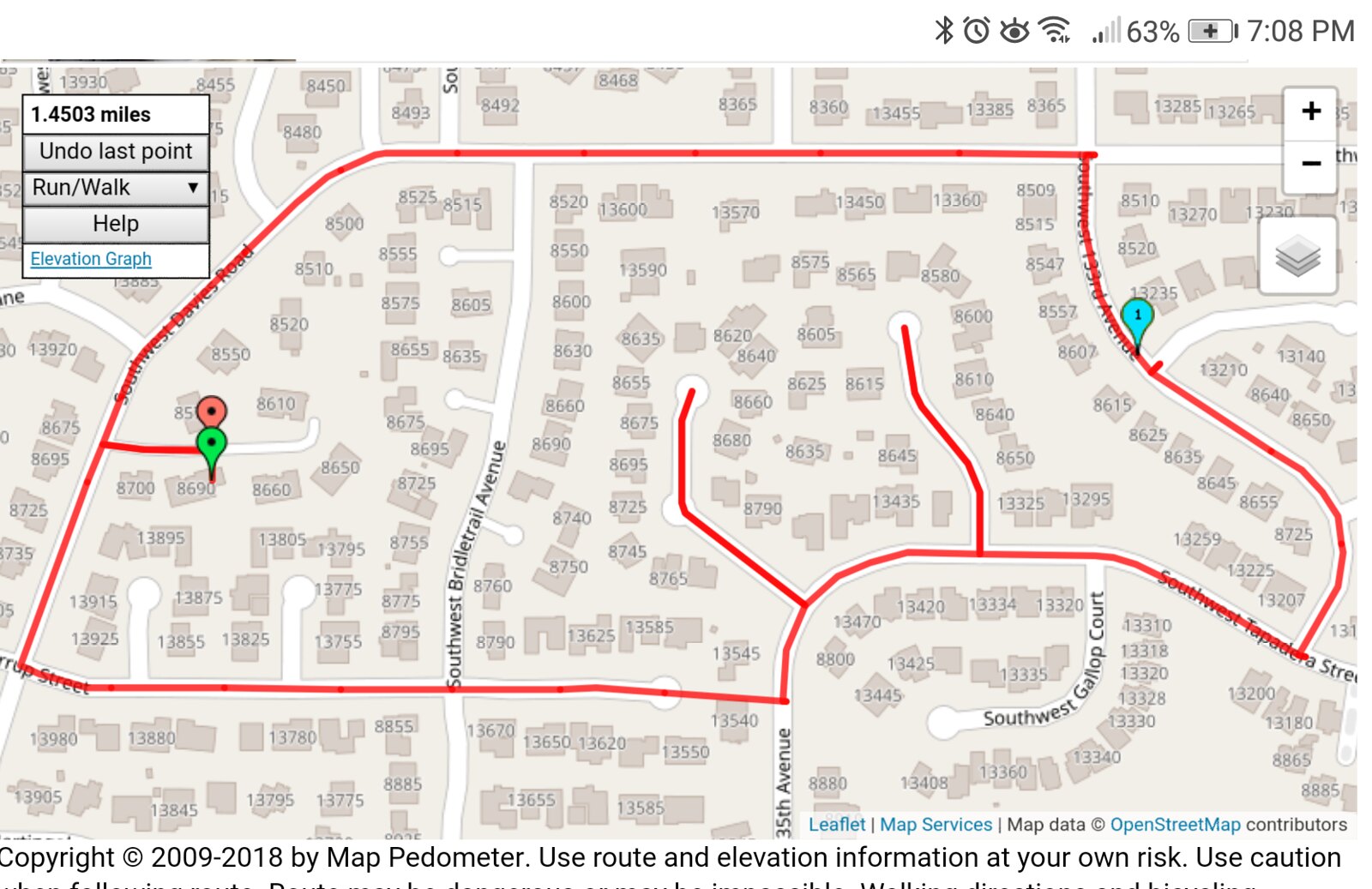This image is a screenshot of a run-tracking application taken on a smartphone. The screenshot, captured at 7:08 PM, shows a map with tan-colored terrain and white lines demarcating roads. Various houses and buildings are indicated by numbers throughout the map. 

The phone's status bar is visible at the top, displaying the time, battery level at 63%, and some icons and notifications. In the top-left corner of the screen, a drop-down menu is available for marking points, undoing points, or setting the session as a run or walk. The top-right corner features zoom in and zoom out buttons.

The map itself includes several points marked in different colors: one red, one green, and one teal blue. A red line illustrates the route the user is likely running. At the bottom of the map, there is copyright information attributed to 'per domitor.'